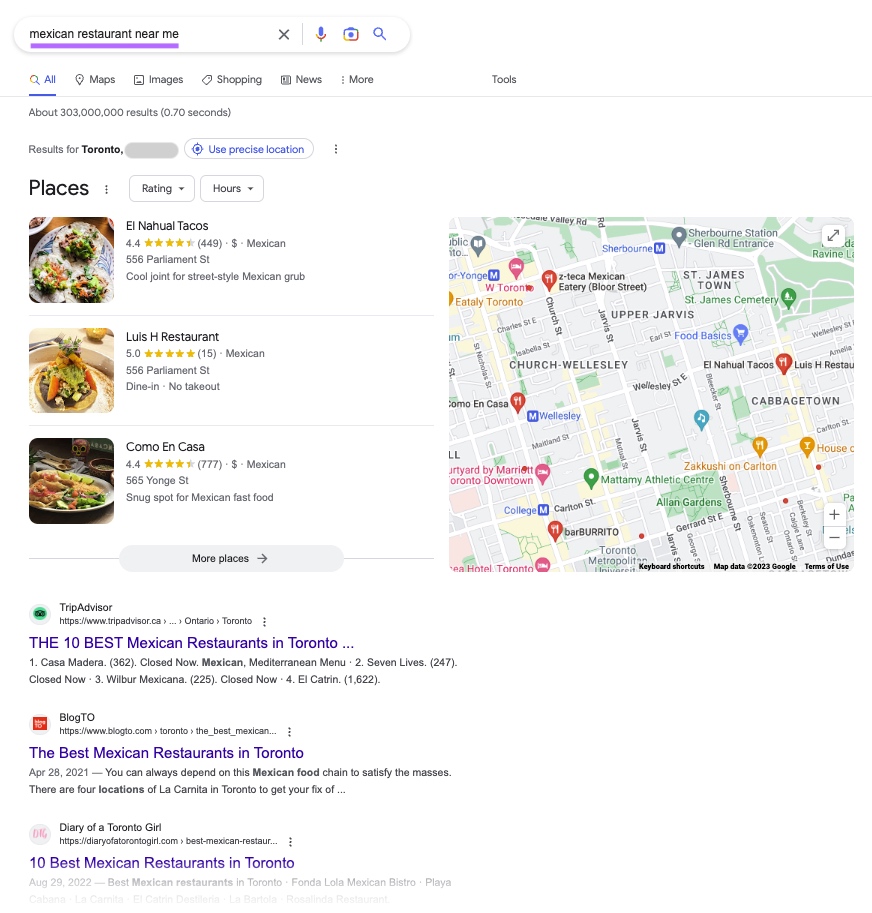The image is a screenshot of a Google search query for "Mexican restaurants near me," likely conducted in the Toronto area. The search interface displays familiar categories at the top such as 'All', 'Maps', 'Images', 'Shopping', 'News', 'More', and 'Tools,' with 'All' being highlighted in blue and underlined, indicating it's the active tab.

The results highlight three Mexican restaurants: El Nahuel Tacos, Luis H. Restaurant, and Como en Casa. Accompanying these entries are thumbnail images of Mexican dishes that resemble tostadas, salads, and tortillas, although the exact food items are indistinguishable. Each restaurant entry includes a star rating, addresses, and options for dine-in or takeout.

Below the initial listings, a section in gray labeled "More places" includes additional options. These entries lead to external sources such as TripAdvisor, which lists the "10 Best Mexican Restaurants in Toronto." The top three restaurants on this list are Casa Madera (currently closed), Seven Lives (also closed), and Wilbur Mexicana (closed as well). Another source is BlogTO, which compiles a similar list of the best Mexican eateries in Toronto. Lastly, the site "Diary of a Toronto Girl" features an article titled "10 Best Mexican Restaurants in Toronto."

Overall, the screenshot captures a detailed snapshot of Google search results for Mexican dining options in Toronto, encompassing user ratings, operational statuses, and expert recommendations.